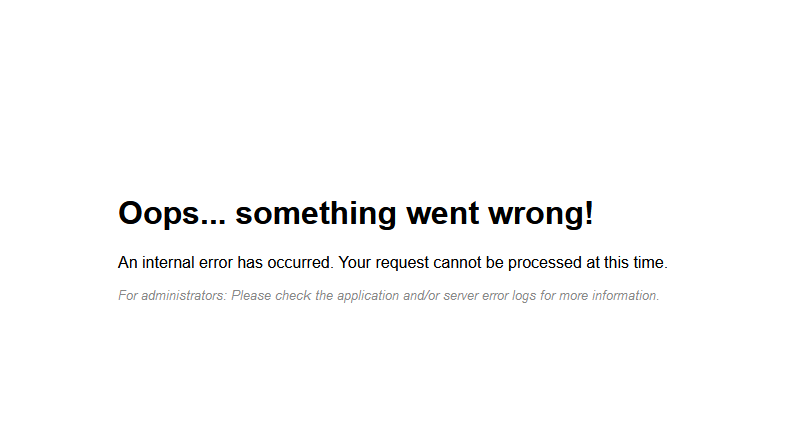**Detailed Screenshot Description: Error Page**

The screenshot captures an error page that appears when a website encounters an issue. The message is displayed prominently in black text against a blank white background, contributing to the stark and uncompromising nature of the error notice.

At the top, the message "Oops... Something went wrong!" is written in bold black letters, immediately drawing the viewer's attention to the problem. Below this, in smaller black text, the page elaborates, stating: "An internal error has occurred. Your request cannot be processed at this time." This message indicates that the problem is server-related and not a fault of the end-user.

Further down, in even smaller gray text, a more technical message appears for site administrators: "For administrators: please check the application and/or server error logs for more information." This suggests that the issue could be diagnosed and hopefully resolved by inspecting server logs.

The rest of the screen remains entirely blank, providing no additional context about the website's identity or the user's intended activity. There are no visible tabs, navigation buttons, or mouse cursors on the screen, making it impossible to determine which website the error occurred on.

This type of error message is typically displayed when a website experiences significant technical challenges, such as high traffic volumes overwhelming the server, connectivity issues, or other internal malfunctions. The clean layout of this error page makes its message clear and unambiguous, but offers little comfort or action steps for the user.

In summary, the image reflects a typical scenario where the website fails to handle a user's request, displaying a clear but uninformative error page that leaves the user unable to proceed with their intended task.